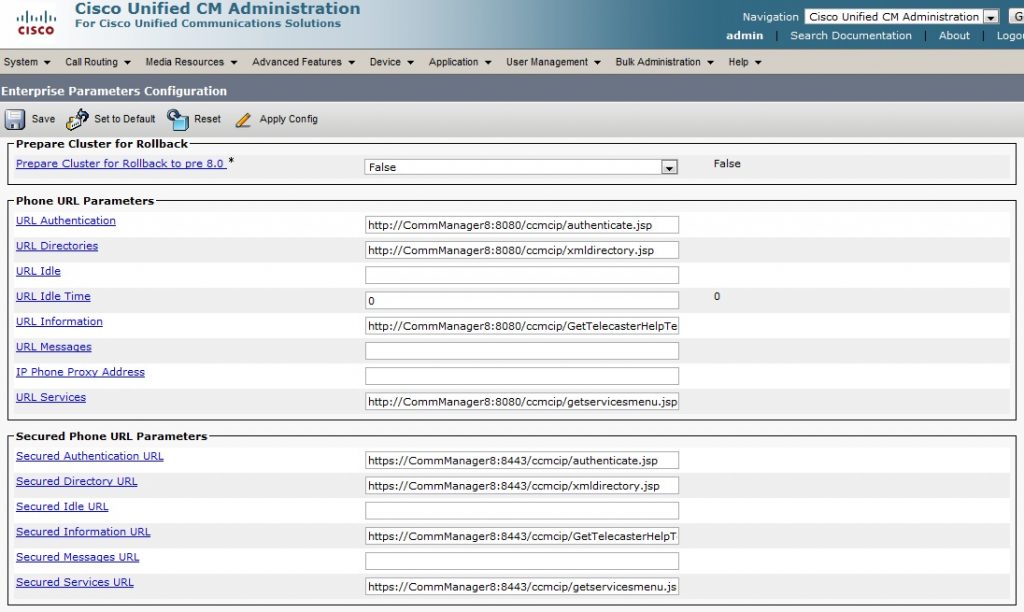This is an image of a Cisco Unified CM Administration webpage, part of the Cisco Unified Communication Solution. The top portion of the page has a blue banner with white text that reads "Cisco Unified CM Administration" and features the Cisco logo on the left. To the right, there is a navigation section labeled "Navigation" with a drop-down menu displaying "Cisco Unified CM Administration."

Below this, there is a secondary navigation bar in gray with black text and drop-down arrows for various categories. These categories include System, Call Routing, Media Resources, Advanced Features, Device, Application, User Management, Bulk Administration, and Help.

A section labeled "Enterprise Parameters Configuration" in gray contains several icons: a save icon (depicted as a disk), a "Set to Default" icon, a reset icon, and an "Apply Config" icon.

The main content is divided into three outlined sections:

1. **Prepare Cluster for Rollback**
   - Title: "Prepare Cluster for Rollback to pre 8.0" (with an asterisk)
   - Center Field: "FOSS"
   - Right Field: "FOSS"

2. **Phone URL Parameters**
   - URL Authentication: `http://commanager8:8080/CCMCIP/authenticate.jsp`
   - URL Directories: `http://commanager8:8080/CCMCIP/XMLDirectory.jsp`
   - URL Idle: (Field is empty)
   - URL Idle Time: (Fields are both 0)
   - URL Information: `http://commanager8:8080/CCMCIP/getTelecasterHelpTE...` (text cut off)
   - URL Messenger: (Field is empty)
   - IP Phone Proxy Address: (Field is empty)
   - URL Services: `http://commanager8:8080/CCMCIP/getServicesMenu.jsp`

3. **Secured Phone URL Parameters**
   - Secured Authentication URL: `http://commanager8:8080/CCMCIP/authenticate.jsp`
   - Secured Directory URL: `http://commanager8:8080/CCMCIP/XMLDirectory.jsp`
   - Secured Idle URL: (Field is empty)
   - Secured Information URL: `http://commanager8:8080/CCMCIP/getTelecasterHelpTE...` (text cut off)
   - Secured Messages URL: (Field is empty)
   - Secured Services URL: `http://commanager8:8080/CCMCIP/getServicesMenu.jsp`

Each section title is in black and the options within each section are blue and underlined, suggesting they are clickable links or fields. The layout indicates an organized interface for managing various configurations and settings for Cisco's Unified Communication services.